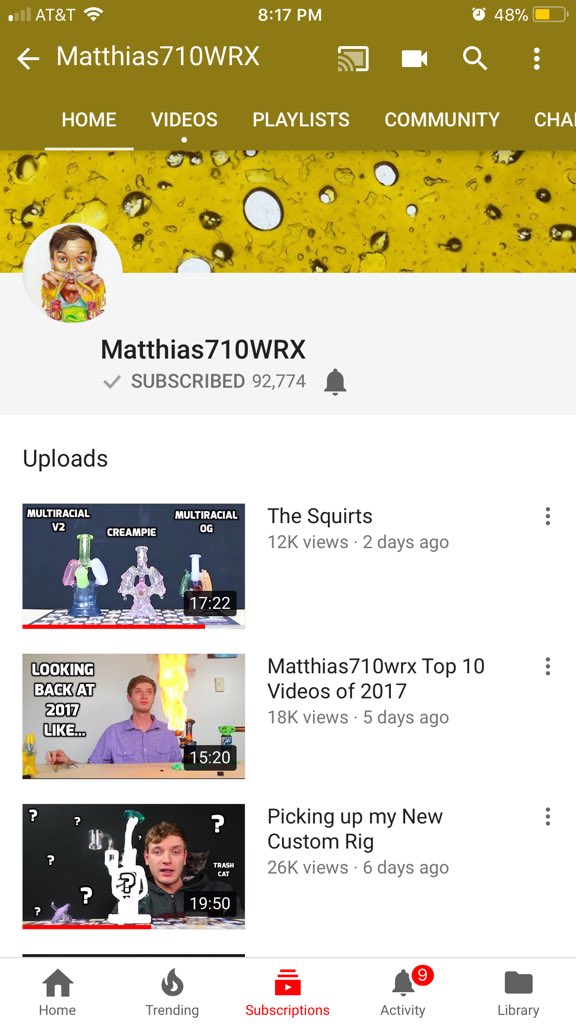A detailed screenshot of a mobile phone screen is captured in the image. At the top, there is a distinctive tan mustard-colored notification bar showing one Wi-Fi bar with AT&T service, an 817 p.m. timestamp in the center, and a Wi-Fi signal icon to the right. The battery indicator on the far right shows 48% remaining. Just below this status bar, "Matthias 710 WRX" is displayed in white text.

Next, there is a navigation bar containing a cast icon, a movie icon, a search icon, and three vertical dots for additional options. Beneath this bar, another menu strip includes tabs titled "Home," "Videos," "Playlist," "Community," and a partially visible tab to the far right.

A prominent banner image spans the width of the screen, featuring a pattern resembling yellow and white elements under a microscope. To the left of this banner, there’s an icon of a man’s face wearing a multicolored shirt, which suggests a Facebook profile picture. Next to the icon, "Matthias 710 WRX" is displayed in black text with subscriber count of 92,774.

Below these details, Matthias’ video uploads are listed. The first video is titled "The Squirts," followed by "Matthias 7110 WRX Top 10 Videos of 2017," and "Picking Up My New Custom Rig." Each title is accompanied by a relevant thumbnail image to the left.

At the bottom of the screen, there are navigation icons for "Home," "Trending," and "Subscriptions" in brown and gray, positioned in the center. On the right side, there is a gray activity bell icon with nine notifications and a gray library file folder icon.

The image captures a detailed view of Matthias 710 WRX's online presence, showcasing his videos, subscriber count, and user interface details relevant to the application being used.